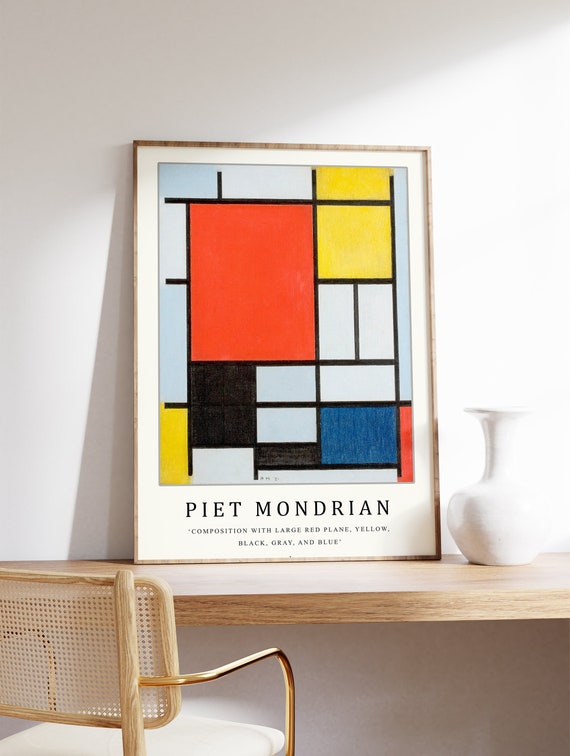The image features a framed modern art poster by Piet Mondrian, identifiable by the thin brown frame with a white border. The text at the bottom reads "Composition with Large Red Plane, Yellow, Black, Gray, and Blue." The artwork displays Mondrian's signature style with variously sized squares and rectangles in colors such as blue, red, yellow, black, and gray. The framed poster is leaning against a white wall, casting a shadow across the scene. It is placed on a light wooden table, atop which also sits a white vase without flowers. To the left of the scene is a chair with a white cushioned seat, a mesh back, and gold metal arms. Light from a window to the right illuminates the room subtly.